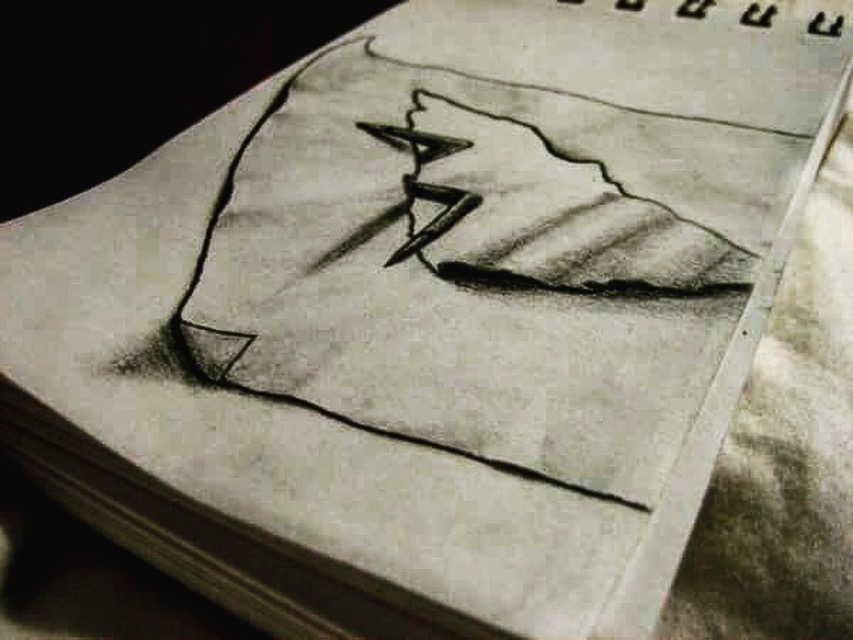A monochromatic photograph captures an open sketch pad laid flat, with its top page displaying an intricate, hand-drawn illustration. The artwork on the page features a rectangular shape, meticulously rendered in pencil, with one corner artistically curled upwards, giving the impression of an ancient scroll or parchment turning up. The realistic shading enhances this three-dimensional effect. Inside this cleverly drawn frame, a mysterious image emerges, dominated by forms resembling an 'M' and a triangular structure. The interplay of light and shadow within the drawing hints at a combination of ink and pencil mediums. The captivating simplicity of the sketch pad against the stark black and white palette invites the viewer to ponder the story behind the unfinished artwork.